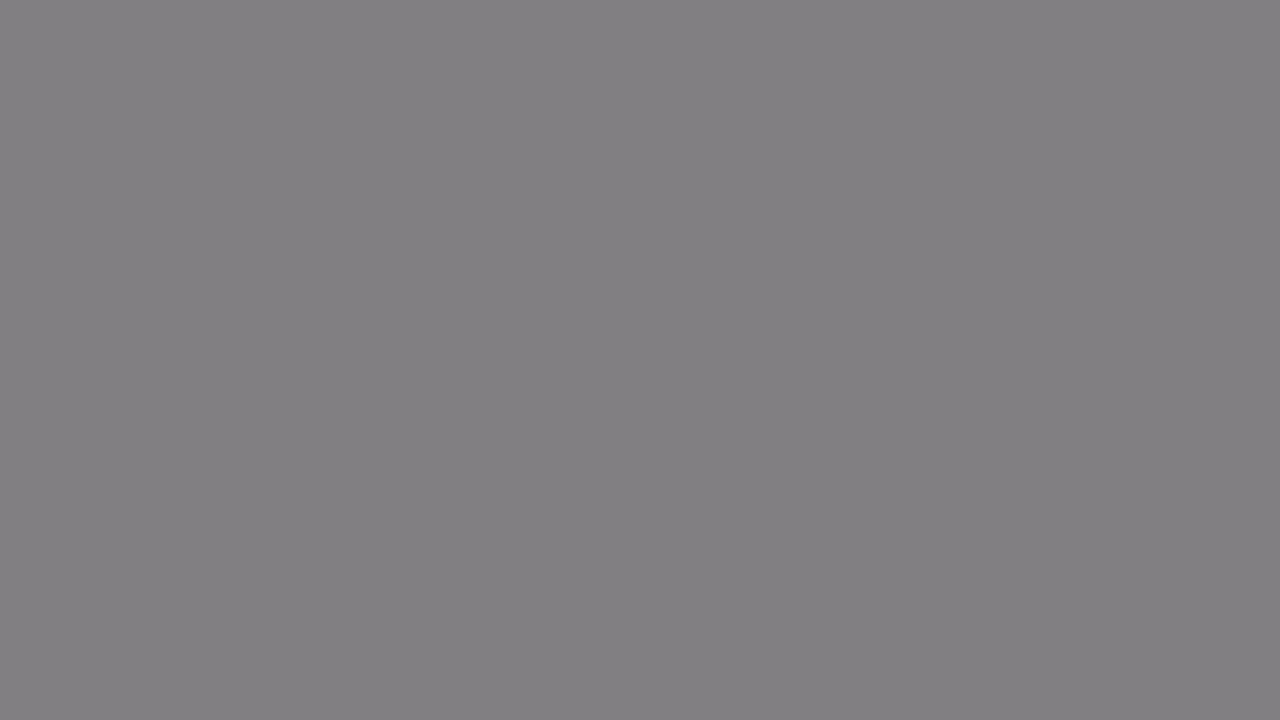The image depicts a simple, plain gray square with a consistent dark charcoal gray tone. The entire image is uniformly colored, with no varying shades or gradients. There are no objects, text, or distinguishing elements in the composition. It is a flat, unaltered background that occupies the whole frame, remaining consistent and unchanging across the top, bottom, left, right, and center. This solid gray color dominates the entire image without any hint of foreground or background differentiation.